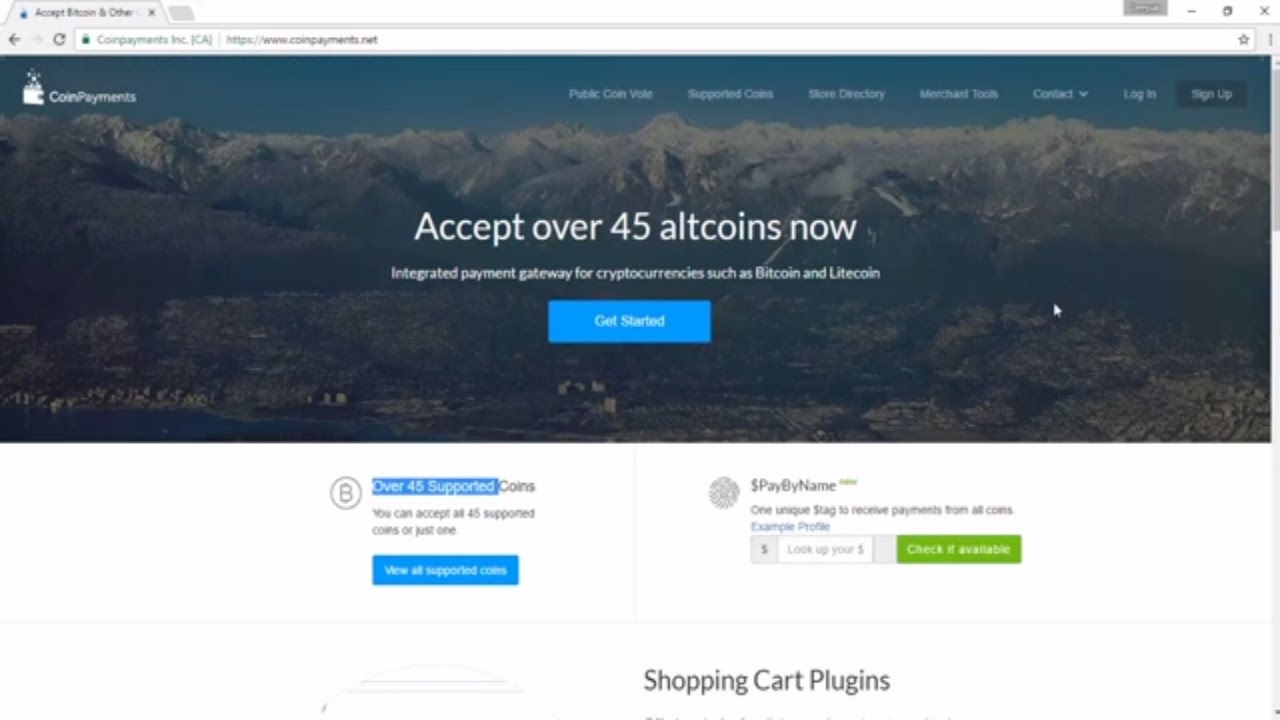Screenshot of a website in landscape mode, featuring a light gray top bar. The top left corner has an unreadable tab, while the top right displays various action icons, including an 'X' for closing the page, and other icons possibly for zoom and expand functions. Below the gray bar is a long white search bar with a padlock icon, containing a secure HTTPS URL for "coinpayments.net."

A panoramic photograph of an arid mountain range occupies the central section of the screenshot, with the "CoinPayments" logo—depicted as a white icon resembling coins dropping into a jar—situated in the top left corner. 

On the right side of the image are 'Login' and 'Sign Up' buttons, accompanied by five menu options on the left, with 'Contact' being one of them and featuring a dropdown arrow. The remaining menu options are too small to read.

Overlaying the photograph, large white text reads: "Accept over 45 altcoins now. Integrated payment gateway for cryptocurrencies such as Bitcoin and Litecoin." Below this is a bright blue horizontal rectangle with the text "Get Started."

Beneath the panoramic image, the bottom section features a white space with truncated content, including the partially visible text "Shopping cart plugins" and a vertical scroll bar indicating there is more content below.